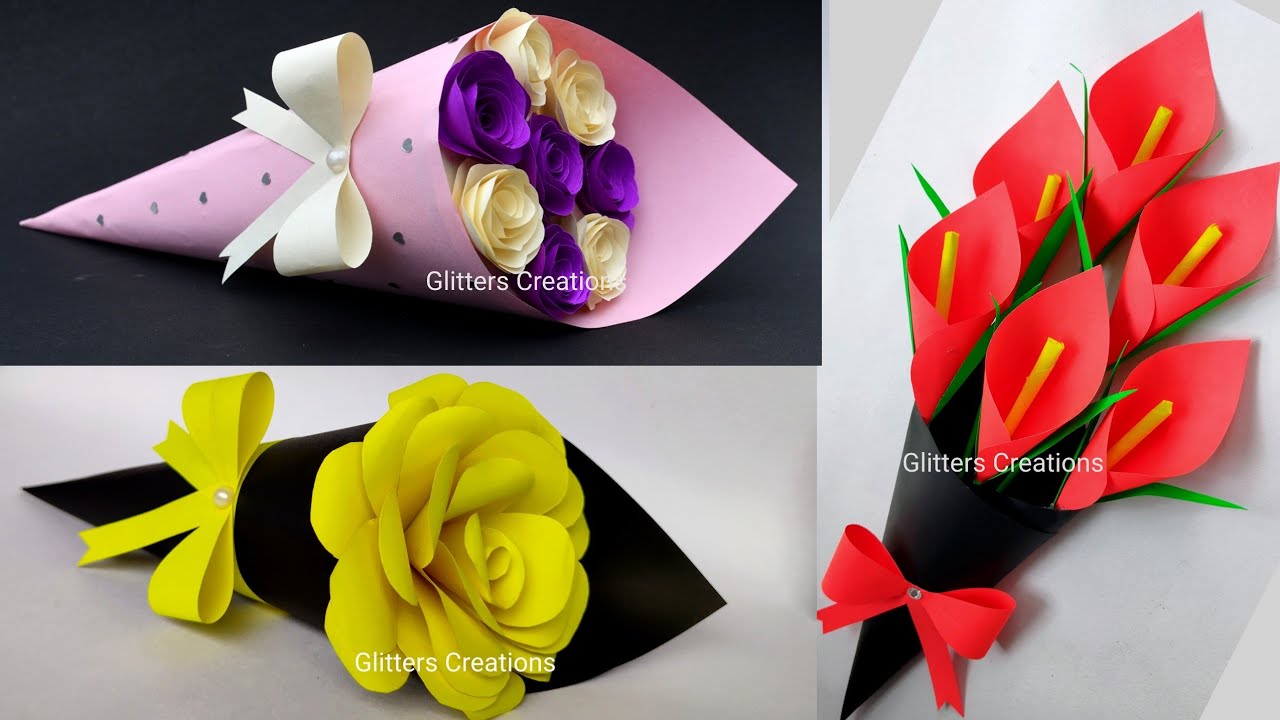The image consists of three distinct, color-saturated photographs arranged in a landscape orientation, each capturing paper-crafted flowers housed in decorative paper cones associated with the brand "Glitters Creation." The top left photograph features a lavender cone adorned with a white ribbon in the middle, containing eight paper roses—four dark purple centered and two cream-colored roses positioned at the top and bottom, all set against a black background. The text "Glitters Creation" appears in white at the top. Below this, on the bottom left, is a photograph of a black paper cone lying sideways, showcasing a single large yellow rose secured with a yellow ribbon, also set against a white background with the same white text at the top. The photograph to the right, arranged vertically, displays another cone with a red ribbon tied at the top, holding six conical-shaped red flowers with gold stamens, resembling tropical flowers, and additional green sprigs, all positioned diagonally on a white background, with "Glitters Creation" text in white. The varying backgrounds and compositions are brought together under a coherent thematic presentation of paper-crafted floral arrangements.